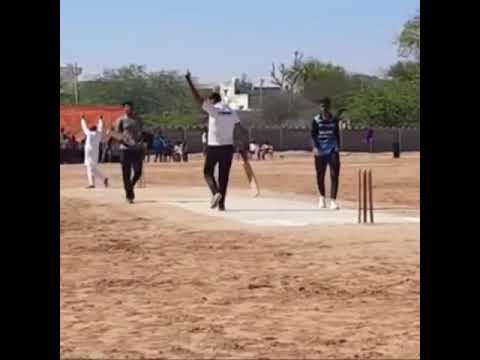The image portrays a sandy, dirt field enclosed by a fence, indicative of an outdoor sporting arena, potentially for cricket, given the presence of the characteristic poles sticking out of the ground. In the center stands a man with darker-toned skin, dressed in a white t-shirt with indistinct writing on the back, black pants, and tennis shoes. His left arm is raised high. To his left, another man in a green shirt, black pants, and tennis shoes gazes off into the distance. On his right, a third man wears a blue and white striped shirt with black pants and white tennis shoes. Additionally, there's a distant figure dressed in full white, also with arms raised. The background reveals a reddish-colored building on the left, a high-rise structure in the middle, and scattered trees. Several small, indistinct figures, possibly spectators, are visible further away, adding to the ambiance of an organized event.